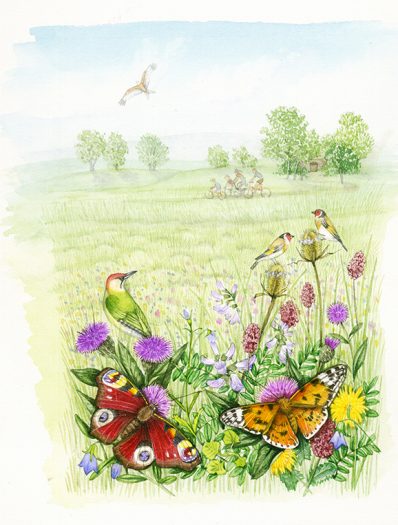This is a detailed portrait format painting of an idyllic outdoor scene. The sky is a light blue with puffy white clouds and features a brown bird flying in the top left corner. Below the sky, the background reveals a mountain range or rolling green hills, with six trees—three large ones on the right and five medium-sized ones on the left. 

In the midground, a family of four bicyclists, two parents and two children, can be seen riding through a manicured meadow. The figures of the cyclists are moving from right to left, with the tallest adult figure in the back.

The foreground is adorned with several colorful flowers, primarily purple with some red and yellow blooms. Perched on these flowers are three birds with green backs and red heads, resembling finches. Amongst the flowers are also two butterflies: one on the bottom left with a striking dark red color featuring yellow and blue accents, and another on the bottom right, orange with a black and white tiger-like pattern.

Overall, the painting captures a vibrant, lively scene rich in natural details and activity, giving a sense of peaceful harmony in an outdoor setting.